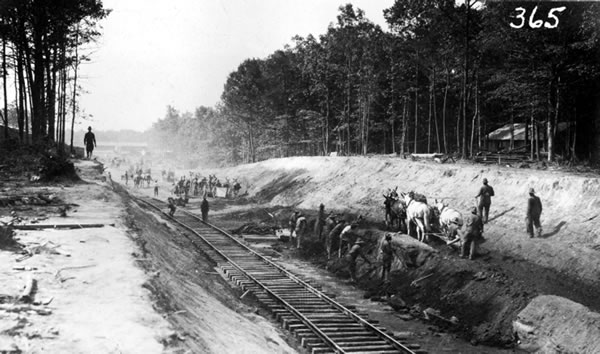This historic black and white image depicts a large-scale construction scene of a railroad track cutting diagonally from the bottom right to the top left of the frame, extending into the distance. The landscape shows embankments on either side where the earth has been excavated. Workers are scattered across the scene, predominantly on the right side where they appear to be laboring in a deeper trench. Among them, several individuals are seen digging and supervising, with some dressed in suits or uniforms and wearing hats. These supervisors stand in contrast to the laborers, creating a dynamic hierarchy within the frame.

In the central right portion, a man guides a cart pulled by white horses, seemingly plowing through the earth. On the right side, near a row of dark-colored, towering trees, more workers appear engaged in their tasks. A faint fog hangs in the center-left background, lending an atmospheric depth to the distant horizon where additional trees and a hill are faintly visible. Overall, the photograph evokes a sense of industrious effort and captures a moment of significant development in the early days of railroad expansion.